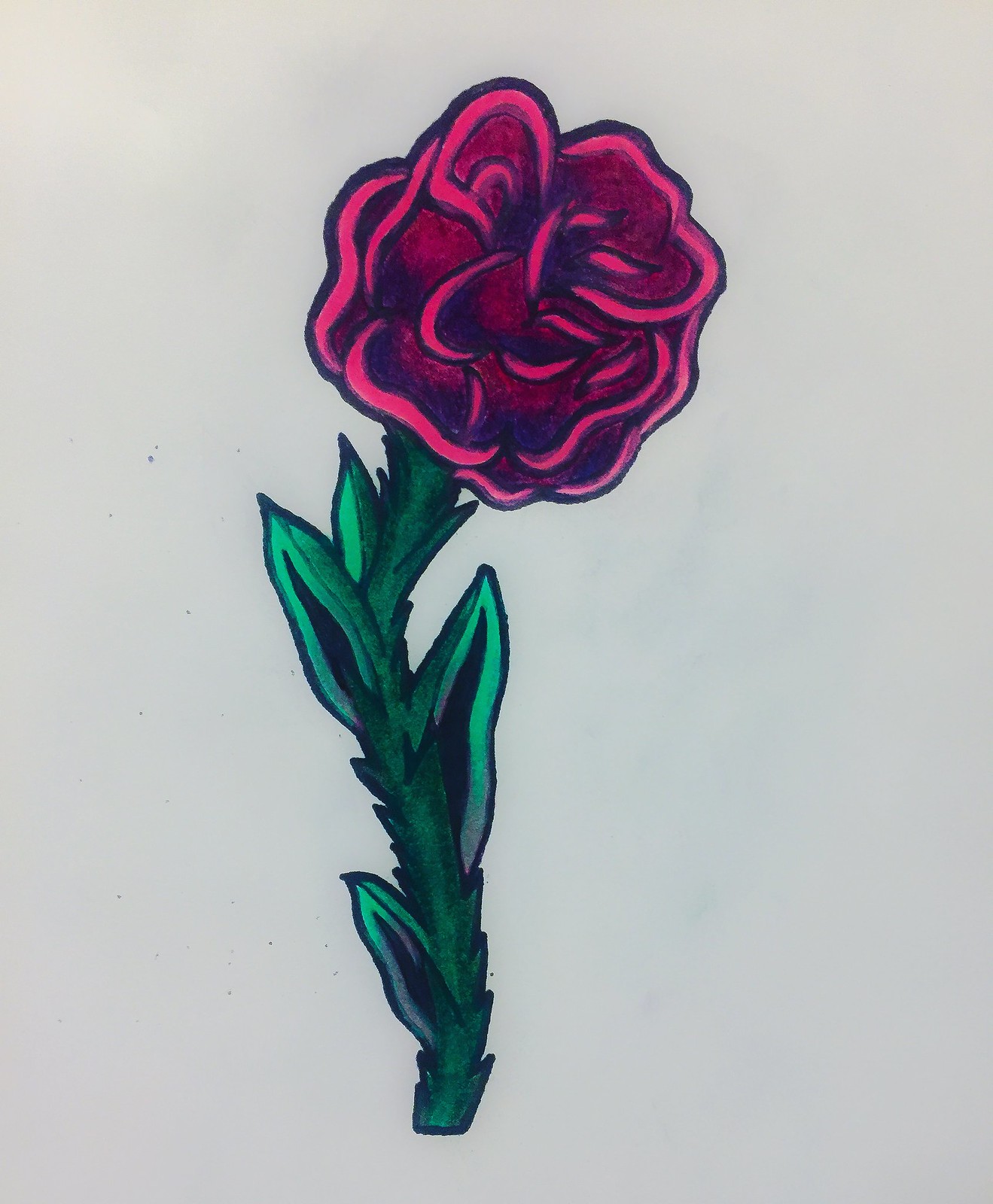This image is a highly detailed drawing resembling a rose, created with Magic Markers on what appears to be beige-cream-white canvas. The multi-petaled flower is vibrant with varying hues, predominantly red with dark maroon outlines accentuating each petal. The petals themselves have a complex color gradient, featuring maroon insides, transitioning through pink, and culminating in a brilliant, almost neon red. Each petal is meticulously outlined, creating a striking, almost ear-like appearance. The thick, straight stem is a rich green, punctuated by four or five leaves that display a range of green shades, from light to dark, with some purple accents. The leaves resemble rabbit ears, having a lighter green outline with a darker green interior. There are no thorns visible on the stem, and the overall shading of the rose enhances its vivid and life-like representation.